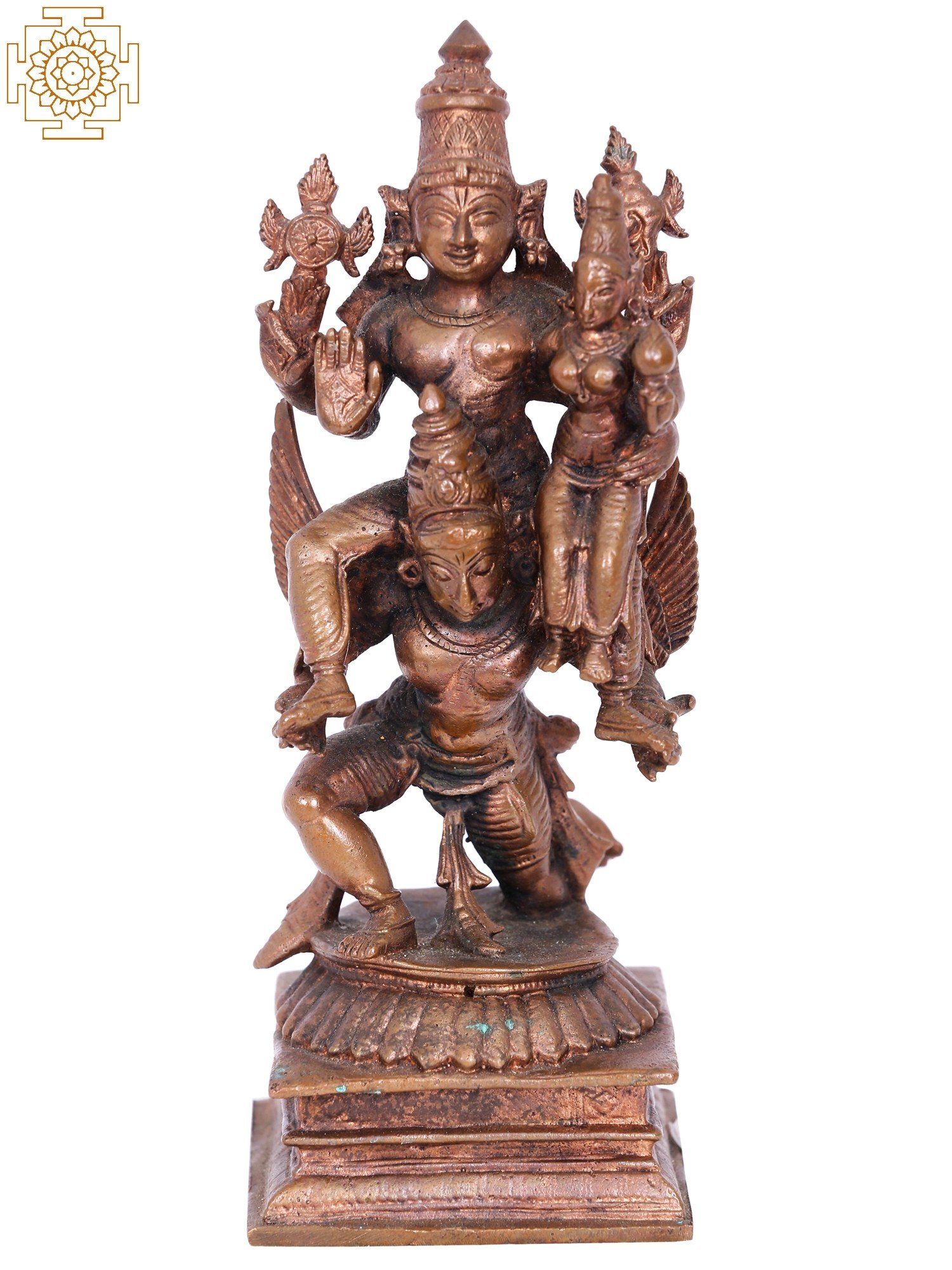The photograph depicts an ancient statue, likely an artifact representing Hindu or Indian deities, crafted in a copper or bronze material with a weathered appearance. Dominating the image is a multi-figured sculpture positioned against a white background. At the monument's foundation is a two-tiered base comprising a circle atop a square. At its pinnacle, a figure, adorned with a tall, intricate headpiece, stands on the shoulders of another kneeling figure, who mirrors the top figure in appearance. The top figure supports a smaller, similarly dressed figure in its left hand. Additionally, a cross-shaped object extends from its right arm. The kneeling figure is depicted with one knee on the ground and the other propped up, and appears to have wings extending from its back. Flanking the scene, in the upper left corner, is a gold symbol: a floral design set within a square frame, adding a decorative touch to the composition.